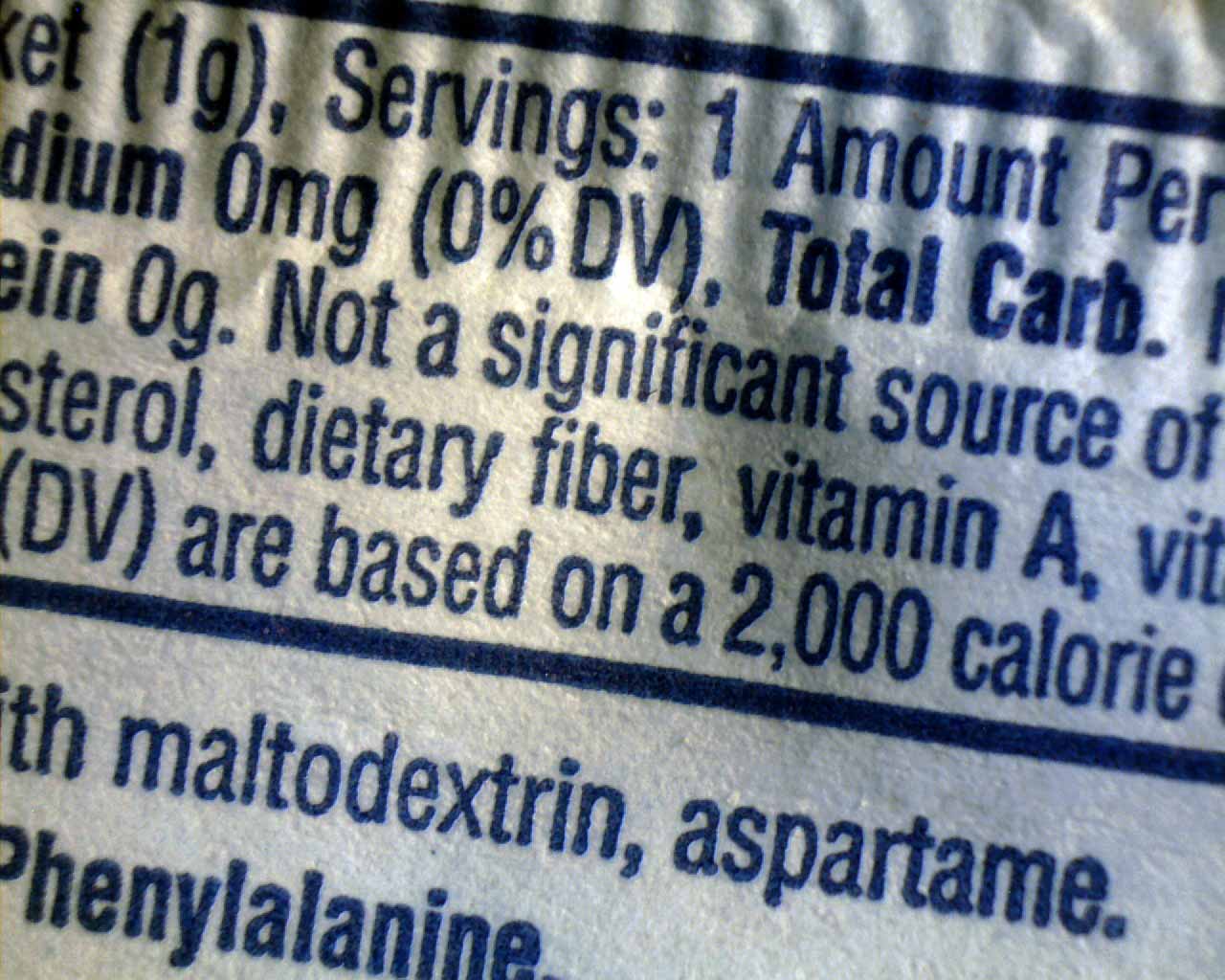This indoor close-up macro photograph captures the details of a nutritional information label. The label, positioned slightly angled to the right, is set against a white background with clearly legible dark blue text. The first line at the top states "servings: 1 amount per," followed by a detailed breakdown of nutrients. "Sodium (OMG) 0% DV," "total carbs," and "not a significant source of" continue in the text, highlighting the limited nutritional content. The label mentions cholesterol, dietary fiber, vitamin A, and emphasizes that "DV are based on a 2,000 calorie" diet. Below a separating blue line, the ingredients list includes "Maltodextrin" and "aspartame." The last line references "Phenylalanine," though the letters are slightly misaligned and tilted downward. The meticulous layout and detailed information make the label's purpose clear, despite some text being partially cut off or slightly distorted.